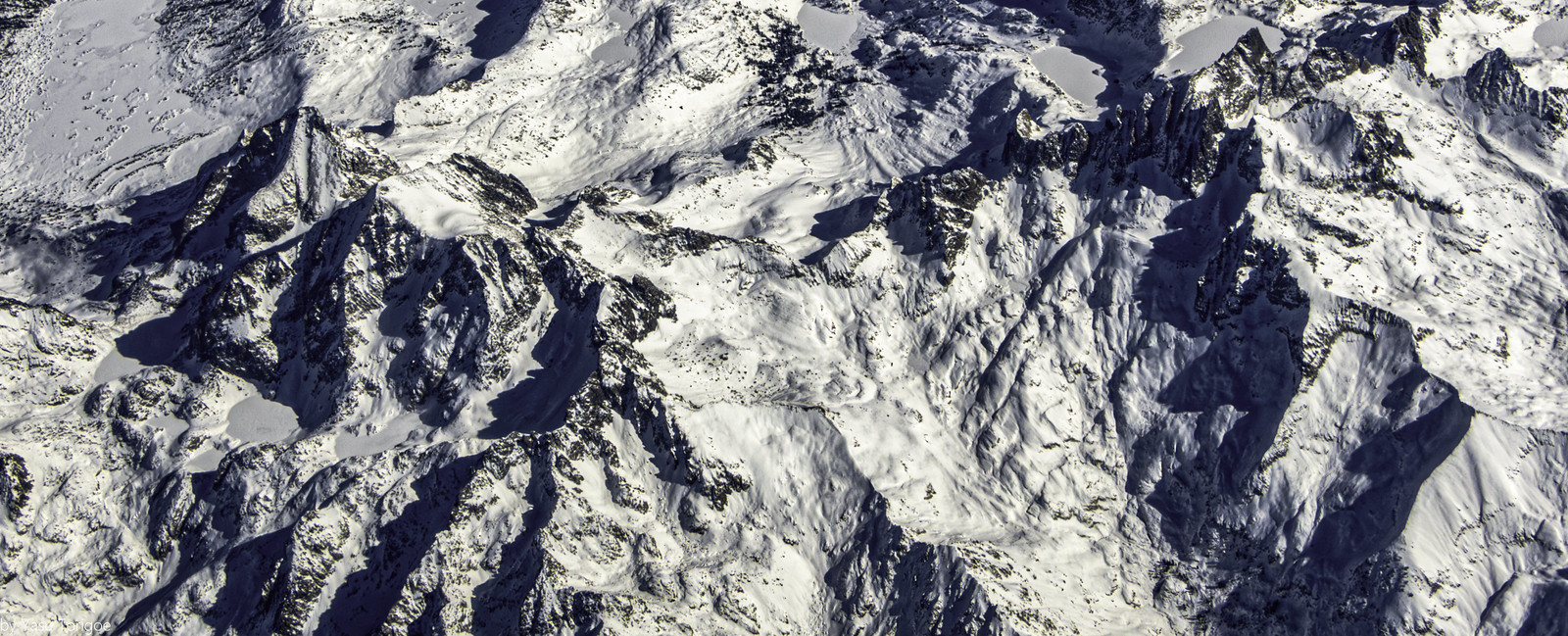This aerial daytime image captures an expansive, snowy mountain range stretching across the frame from the right-hand side towards the left. The scene, viewed from a high elevation almost from the top of the clouds, showcases peaks blanketed in snow but with occasional grayish rocky outcrops protruding through. In the distance on the right-hand side, there appears to be frozen water or ice, adding to the wintry landscape. Moving towards the center of the image, patches of bright blue ocean can be seen in between the mountains, contrasting the predominantly snowy terrain. The entire vista is vast, with the image being about three times as wide as it is tall.